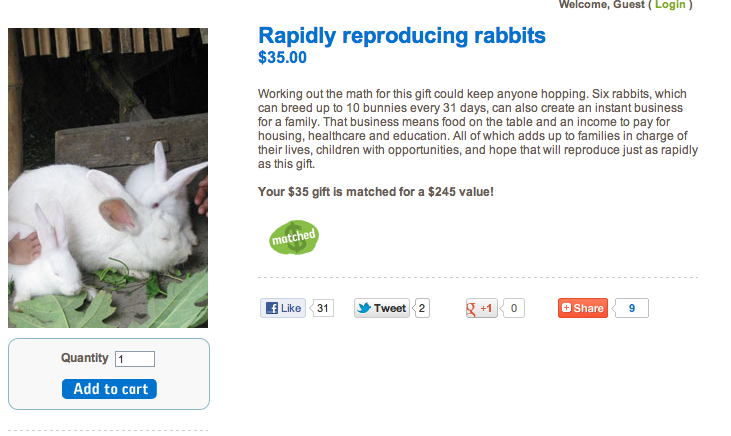"Advertisement for Rapidly Reproducing Rabbits: A vertical photo on the left features three fluffy bunnies with pink ears, nestled among scattered leaves. One rabbit, with its eyes closed, leans forward, while a small and a larger hand gently touch them. The scene is bordered by a wooden bench, serving as a backdrop, and a box displaying the quantity, currently set to one, along with an 'Add to Cart' button in blue. On the right side, in bold blue text, it states: 'Rapidly Reproducing Rabbits, $35.' Above, in the top right corner, are the words 'Welcome, Guest. Log In.' Beneath the price, it reads: 'Working out the math for this gift could keep anyone hopping. Six rabbits, which can breed up to 10 bunnies every 31 days, can also create an instant business for a family.' Additionally, it highlights that a $35 gift is matched for a $245 value. This company offers you the chance to purchase rabbits that, true to their nature, will reproduce rapidly, providing a potential business opportunity."